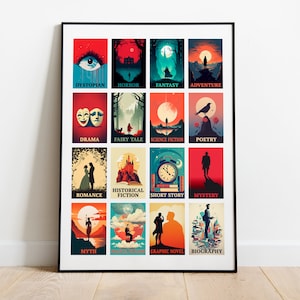The image depicts a large black-framed poster, bordered in white, leaning against a white wall with white trim, resting on a light wooden floor with vertical boards running into the wall. The poster contains 16 squares organized into four rows of four, each square representing a different movie genre. 

Starting from the top left corner, the first row includes:
1. A square featuring an eyeball with a red upper half and blue lower half, labeled "Dystopian".
2. A red and blue-themed square with a mansion, labeled "Horror", displaying a red sky, a moon, and a silhouette walking in the blue-tinged bottom half.
3. A blue and green square labeled "Fantasy", showcasing a fantastical scene.
4. An orange and yellow square with a large moon and a silhouette, labeled "Adventure".

The second row consists of:
1. A square with the drama masks (comedy and tragedy), labeled "Drama".
2. A depiction of Little Red Riding Hood in a forest, labeled "Fairy Tale".
3. An orange square with a large moon and a person walking towards it, labeled "Science Fiction".
4. An image of a bird perched on a mound with a large moon background, labeled "Poetry".

In the third row:
1. A yellow-toned square featuring a couple holding hands, labeled "Romance".
2. A square hinting at a historical setting with what appears to be a castle, labeled "Historical Fiction".
3. A clock encased in a glass dome, labeled "Short Story".
4. A red and black square with a silhouette walking away, labeled "Mystery".

The bottom row includes:
1. A mythical figure holding a long spear in front of a large moon, labeled "Myth".
2. A colorful, aqua-toned square with clouds, contents uncertain.
3. Another square with shadows of people, contents uncertain.
4. A light red and aqua-colored square with confetti-like elements surrounding a person, labeled "Biography".

The light in the room casts a shadow from the right side, emphasizing the left side of the poster.